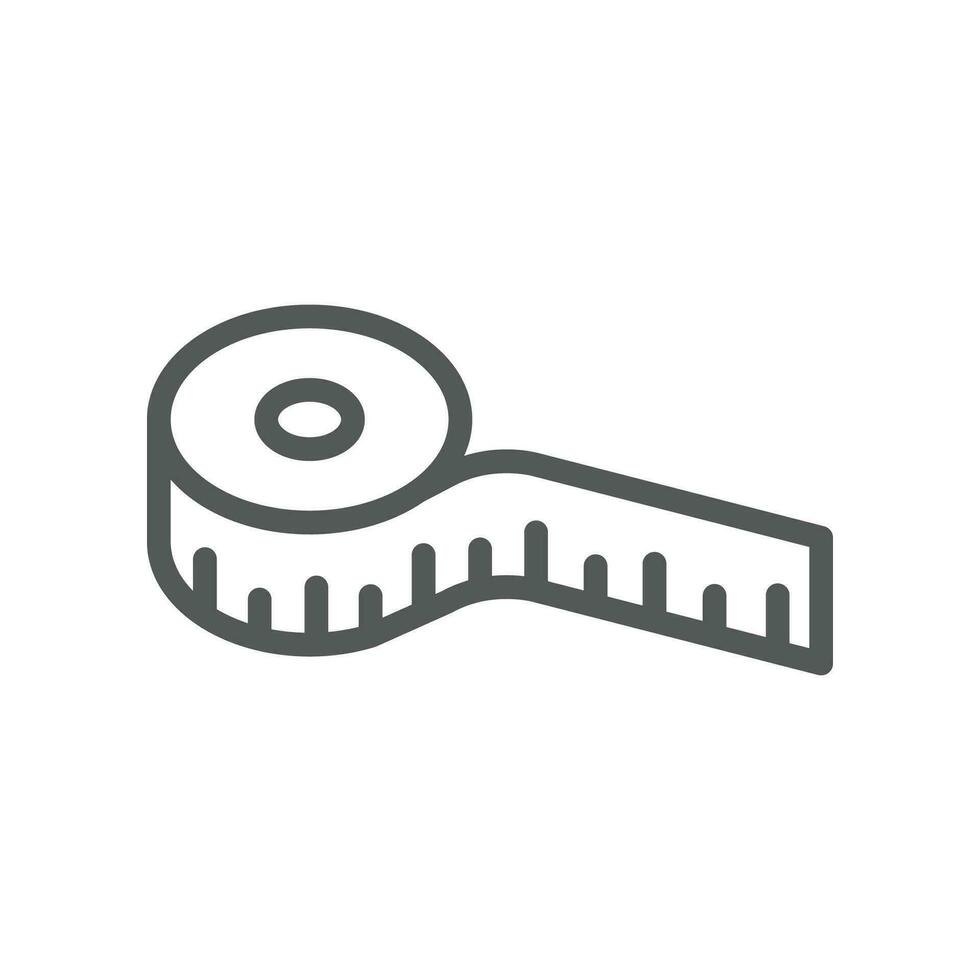The image depicts a highly simplistic and tightly-coiled black-and-white tape measure against a solid white background. The tape measure is circular with an inner hole and is drawn with a continuous, gray line forming both the inner and outer edges of the circle. A short segment of the measuring tape extends straight out from the bottom of the circular coil, featuring additional lines that indicate measurement graduations. The minimalistic design, which could be interpreted as a logo or symbol due to its essential nature, is so straightforward that it could easily be drawn by a child.